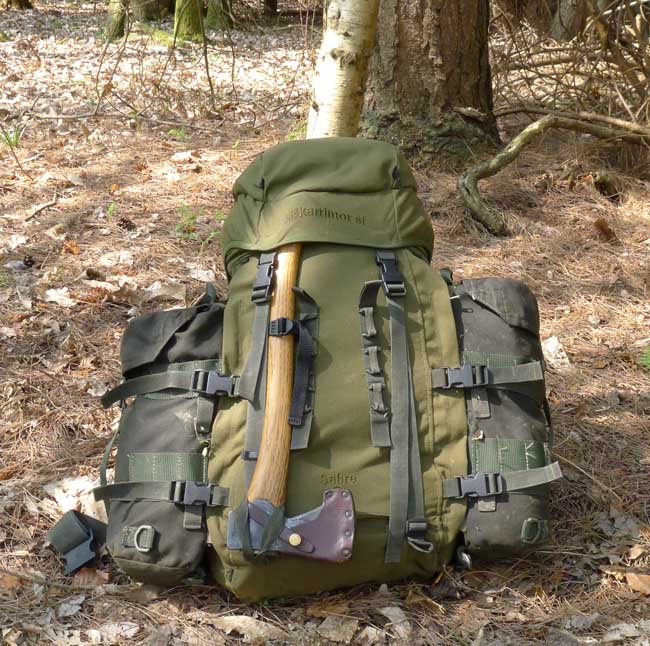The image features an olive green survival backpack resting on a clearing in a wooded area. The ground is covered with brownish pine needles and leaves. Attached to the backpack is an axe with a wooden handle and a reddish-bluish head. The backpack is accompanied by two smaller dark green compartments on either side, providing additional storage. The backpack appears bulky, suggesting it is filled to capacity. In the background, a small tree trunk is visible, with a larger tree trunk further behind, both bathed in sunlight filtering through the canopy.